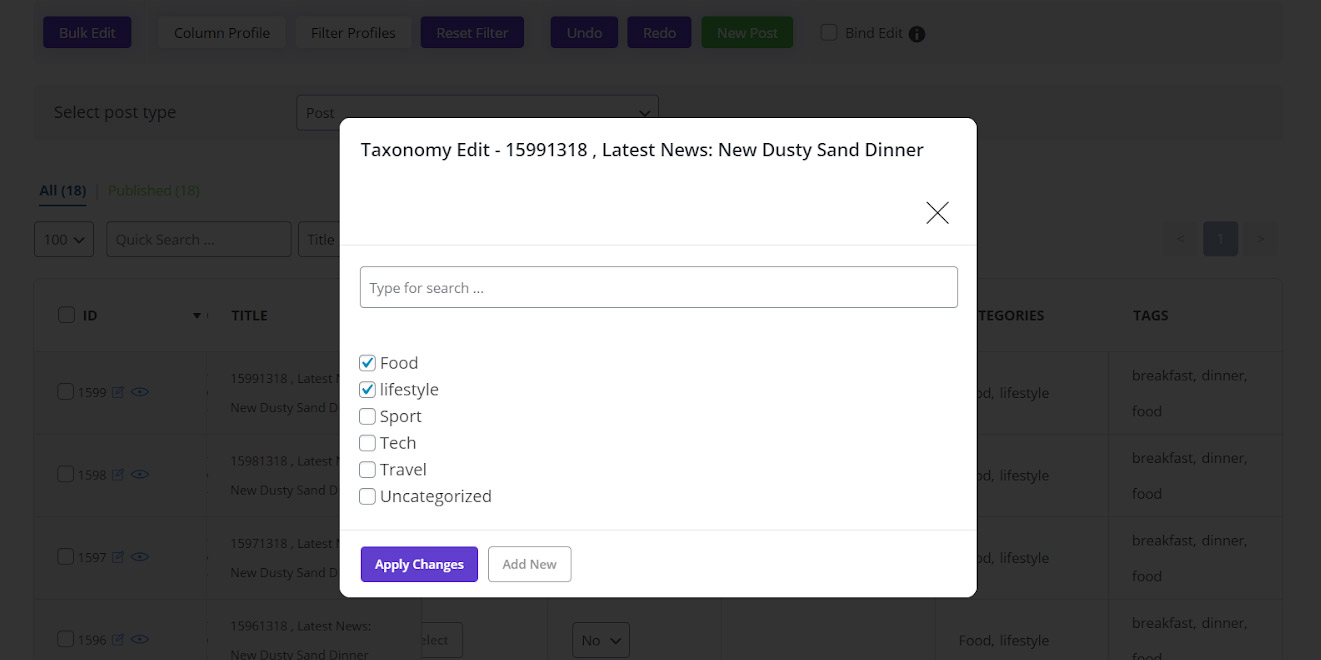Screenshot of a desktop application interface featuring a "Taxonomy Edit" pop-up window. The central white rectangular window, embossed on the screen, is titled "taxonomy edit one five nine nine one three one eight". Below the title is the label "Latest News: New Dusty Sand Dinner." On the lower right corner of this pop-up window, there is a small "X" mark, signifying the close button.

Beneath the title and description, there is an input field labeled "Type for search." Below the search field, there are several checkbox options. The first two options labeled "Food" and "Lifestyle" are checked in blue, while the subsequent options, "Sport," "Tech," "Travel," and "Uncategorized," remain unchecked.

At the bottom of the pop-up window, there is a rectangular purple button labeled "Apply Changes." Adjacent to this button to the right, a link labeled "Add New" is visible.

In the background, behind the "Taxonomy Edit" pop-up, there are various other buttons such as "Bulk Edit," "Profile," "Filter Profiles," "Reset Filter," "Undo," "Redo," and "New Post/Bind Edit," all set against a predominantly dark grey or black interface background, suggesting the focus is currently on the pop-up window in the foreground.